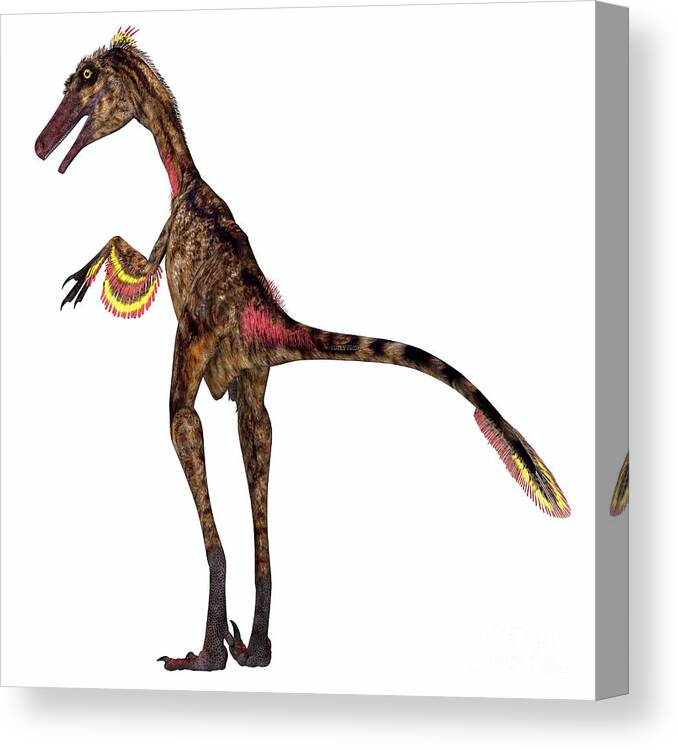This detailed painting of a raptor-type dinosaur dominates a white, 3D canvas that is slightly tilted to the left. Standing on its slender hind legs, the dinosaur's earthy brown skin is interspersed with patches of black, creating a tapestry of browns and darker spots. Its long, narrow tail, adorned with vibrant red and yellow feathering at the end, extends from behind, wrapping partially around the right edge of the canvas. The arms, bent upwards near its chest, also display the same colorful feathering at the elbows. The dinosaur's elongated head, resembling a narrow snout akin to a horse or alligator, features a small mohawk of yellow feathers. Its mouth is open, revealing an absence of visible teeth, while its piercing yellow eye, circled in black, adds to its predatory appearance. The feet and hands are equipped with three sharp, black claws, further emphasizing its raptor characteristics. The overall image exudes a prehistoric and dynamic aura, with the dinosaur captured in a strikingly vivid and lifelike pose.